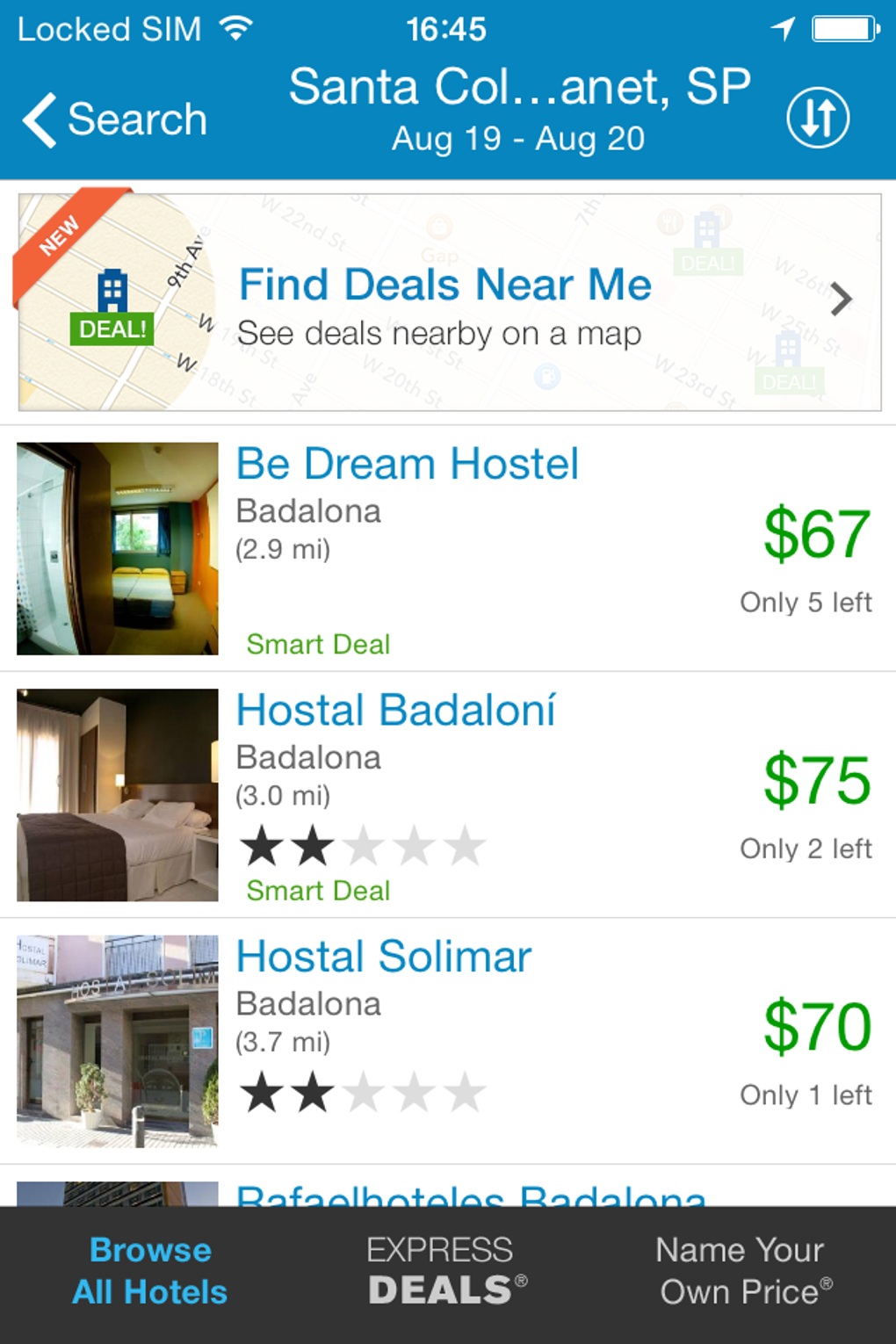At the top of the image, a blue background displays "LOT SIM" in uppercase on the left, followed by the time "16:45" and a full white battery bar on the right. Below this header, the text reads "Santa Col... ANET, SP," with "SP" in uppercase. In the following line, the dates "August 19th through August 20th" are shown, accompanied by a search option to the left.

Below this section, the text "Find deals near me" appears, leading into a list of hostels:
1. **B Dream Hostel in Badalona** (2.9 miles) is listed first. The price is highlighted in green as "$67," with a note to the right indicating there are "only five left."
2. **Hostel Aledona** (3.0 miles) follows, rated two stars out of five. The price, highlighted in green as "$75," mentions "only two left." Additionally, it's marked as a "smart deal."
3. **Hostel Salomar** (3.7 miles) is listed last in this section, also rated with two black stars out of five. The price is shown in green as "$70," with a note explaining "only one left."

At the bottom corner, there's a blue option to "Browse all hotels." In the center, the phrase "Express deals" is displayed, with an option to the right that says "Name your own price."